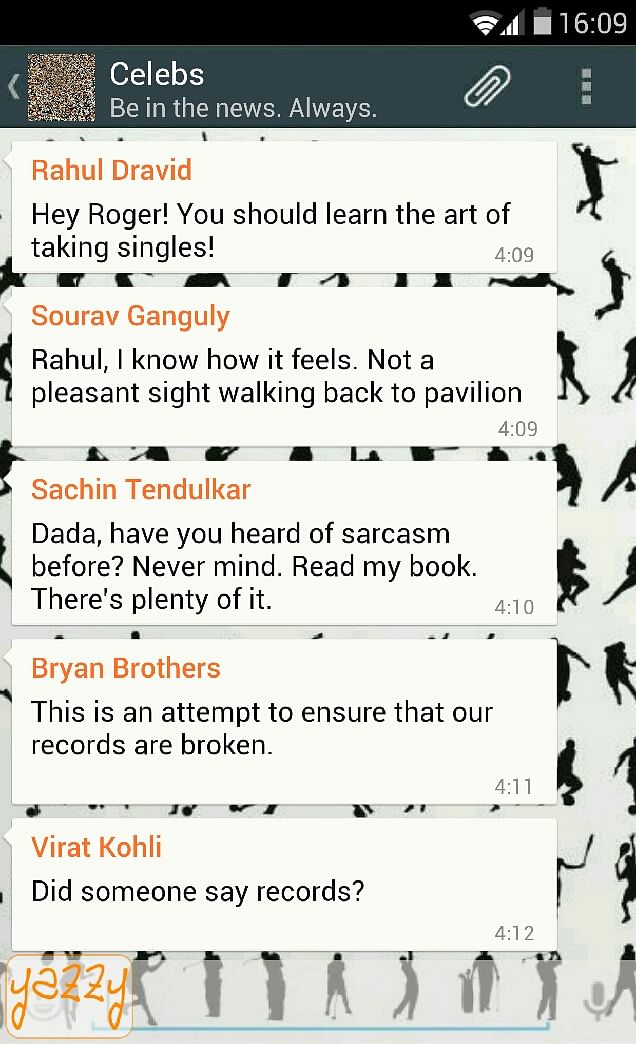The image depicts a cell phone screen featuring a chat interface. In the upper left corner, standard status indicators are visible, including Wi-Fi strength, cellular signal bars, a nearly full battery icon, and the time, which reads 16:09.

The screen displays a series of messages in a group chat titled "Celebs be in the news, always." Below the title, a paperclip icon and a three-squares menu icon are prominently displayed.

The messages include:

1. Ruhul Dravid: "Hey Roger, you should learn the art of taking singles." (16:09)
2. Sourav Ganguly: "Rahul, I know how it feels, not a pleasant sight walking back to the Pavilion." (16:09)
3. Sachin Tendulkar: "Dada, have you heard of sarcasm before? Never mind, read my book, there's plenty of it." (16:10)
4. Brian Brothers: "This is an attempt to ensure that our records are broken." (16:11)
5. Virat Kohli: "Did someone say records?" (16:12)

In the bottom left corner, the name "Yazzy" is highlighted in bright orange with an orange outline, standing out against the background.

The background of the cell phone display features silhouettes of various individuals engaged in different types of sports, adding a dynamic and sporty vibe to the chat interface.